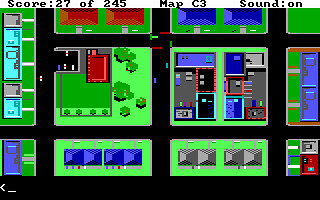The image depicts an overhead view of a computer game set in a neighborhood. The streets are illustrated as black roads, flanked by blocks of houses with green lawns. On the left-hand side, a cluster of blue buildings dominates the scene, interspersed with a few smaller gray structures. At the bottom left, a distinctly darker blue building stands out. Just to its right are a couple of additional blue buildings. Moving upwards, a reddish building is visible, followed by two more reddish buildings further up. To the right of these, two blue buildings come into view, adjacent to a space filled with various colorful elements. This space transitions below into two gray buildings. To their right, a gray building and a red building sit side by side, with two blue buildings positioned above them. Scattered along the roads, small cars add a dynamic element to the otherwise static neighborhood.